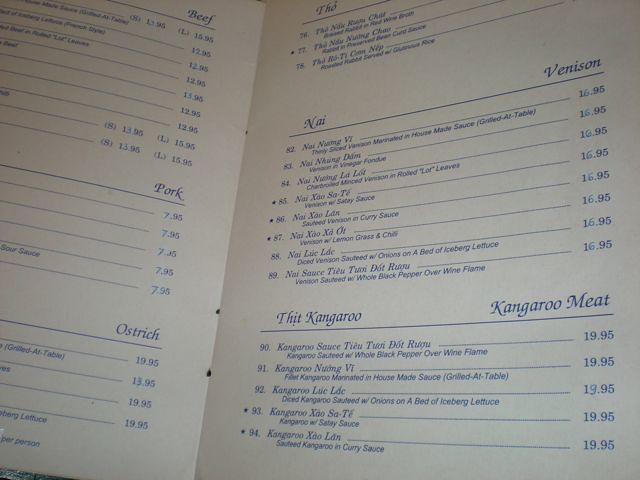This photograph captures a section of a bilingual Vietnamese and English menu, specifically a double-page spread devoted to various meats. In the image, only a portion of the menu is visible. The part of the menu shown includes sections dedicated to beef, pork, ostrich, venison, and kangaroo meat, each titled in both English and Vietnamese. For example, "Thit Kangaroo" is the Vietnamese term for kangaroo meat.

Highlighted dishes under the kangaroo section include "Kangaroo in Satay Sauce" and "Thit Kangaroo Nutmeg V," which is described as fillet kangaroo marinated in house-made sauce and grilled at the table, priced at $19.95. The layout features blue typeface on a white background, and each menu item is numbered sequentially from 76 to 94. Each item's number is accompanied by a star to its left. The detailed presentation ensures clarity for patrons navigating the diverse meat offerings.